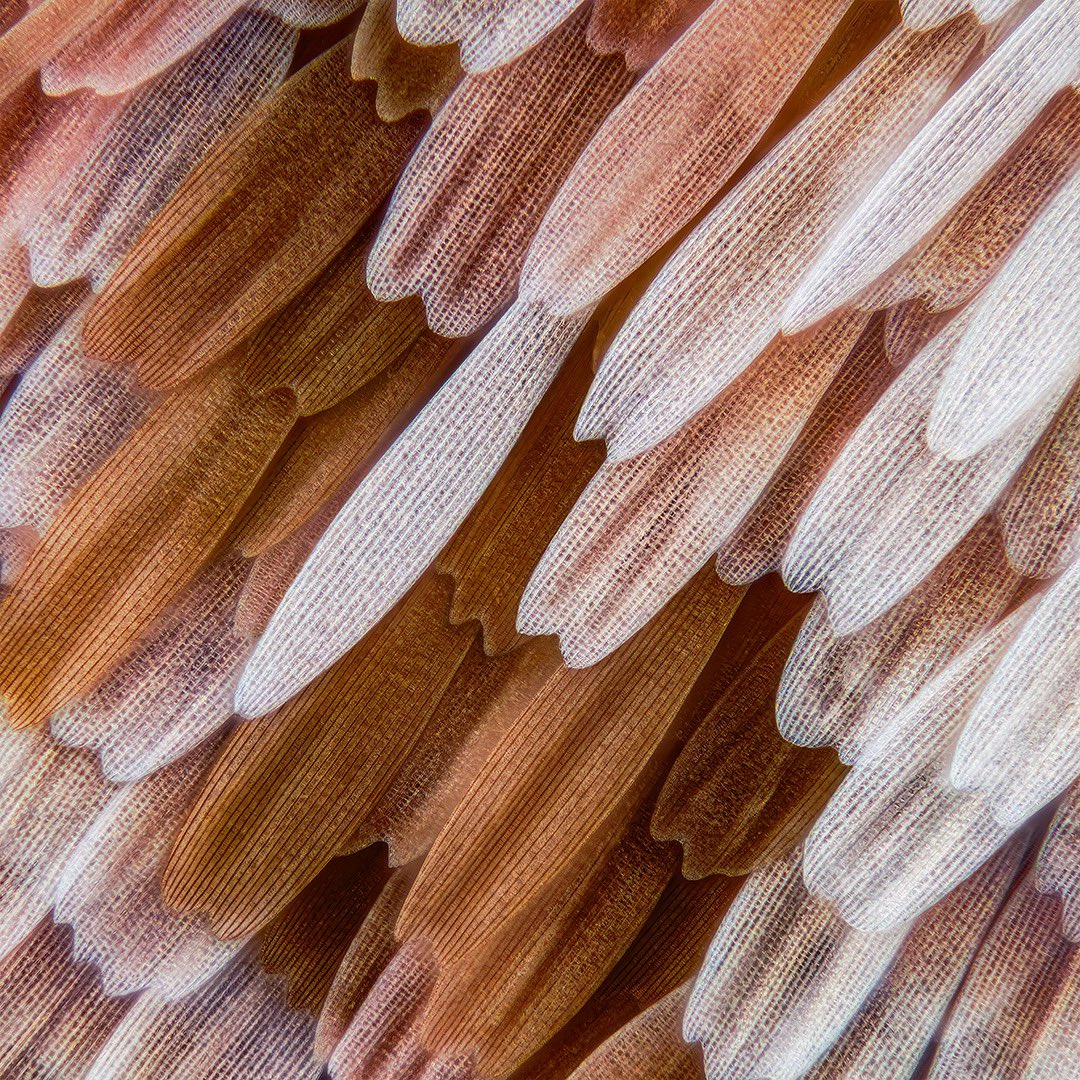The image depicts an extreme close-up view of delicate structures that are difficult to identify definitively. The scene presents an intricate array of layered, almost translucent elements that resemble the petals of a flower, though it's ambiguous whether they may be leaves, fish scales, or fabric weave. The colors are muted and gentle, featuring shades of white, beige, brown, and a touch of soft pink. The structures appear finely detailed, with a hint of a cellular or fibrous texture indicating they could be organic. The delicate elements are layered from the bottom left to the upper right, and the image offers a high level of magnification, making the exact nature of the subject unclear. The subtle interplay of colors and translucency gives the impression of a delicate, possibly natural material viewed up close.